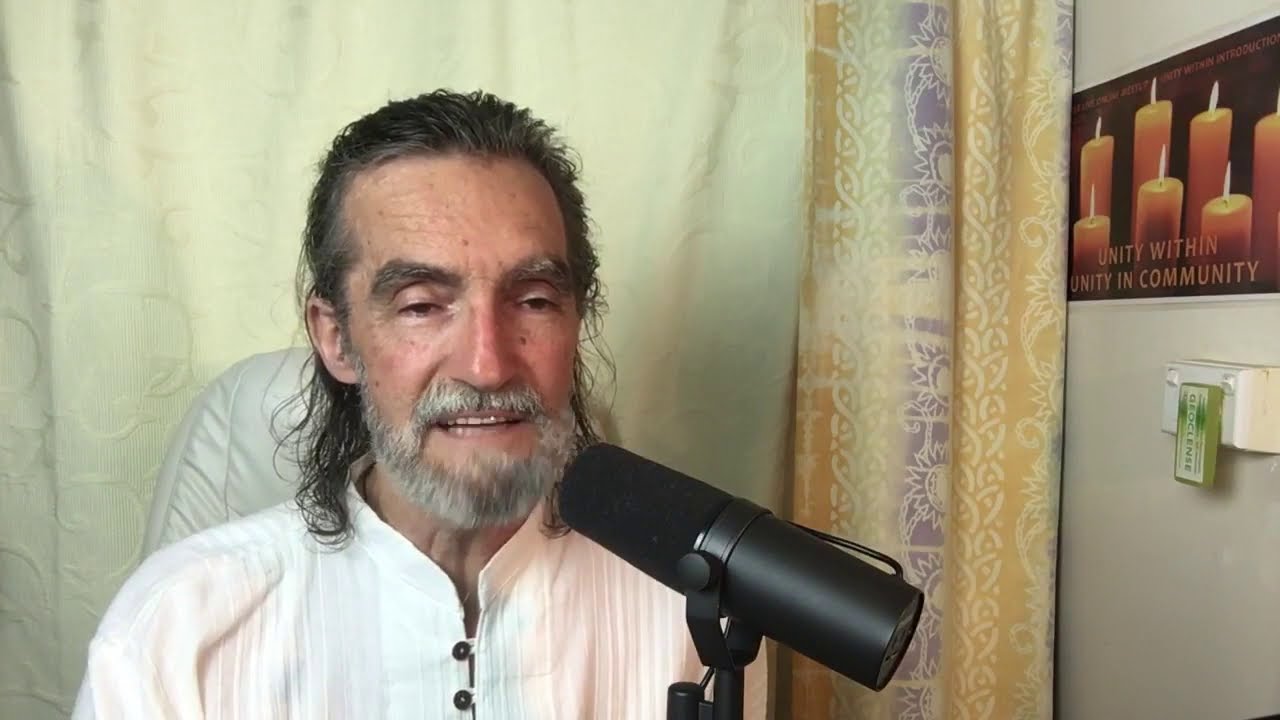This photograph captures an older gentleman, possibly in his mid-50s to 60s, seated indoors. He has a fair complexion, and his hair, a mix of gray and black, is shoulder-length and slicked back. His prominent, bushy eyebrows frame his heavy-lidded eyes, and he sports a thick, white and gray beard and mustache. His mouth is slightly open, revealing his teeth, suggesting he is in the midst of speaking. He is dressed in a light pink shirt with a half collar and is seated in a gray high-backed chair, with the upper part of the chair visible.

Directly in front of him is a large black microphone positioned close to his mouth. The background features a white curtain adorned with decorative yellow and blue borders. To his right, a wall-mounted poster displays images of candles and the words "UNITY WITHIN UNITY IN COMMUNITY," emphasizing a theme of togetherness. Additional details include a possible thermostat device on the same wall. The man's focused gaze suggests he might be speaking into the microphone while engaging with a screen out of frame.